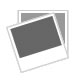The image is a close-up photograph of a gray wool coat draped over a wooden surface, which might also be mistaken for a wall or wardrobe background due to the ambiguity in the positioning. The focus is on the left chest area of the coat up to the neckline. The outer fabric appears rough and dusty, with the color seeming faded, possibly due to the reflection of a bright light source. The coat has big lapels, visible stitching, and a folded outer area. Inside, the coat is smooth with printed patterns and features an additional attachment or strip that can be pulled out. The overall feel of the coat suggests it’s old and in need of a wash, with a worn look enhanced by the grainy wooden or stone-like surface beneath it.